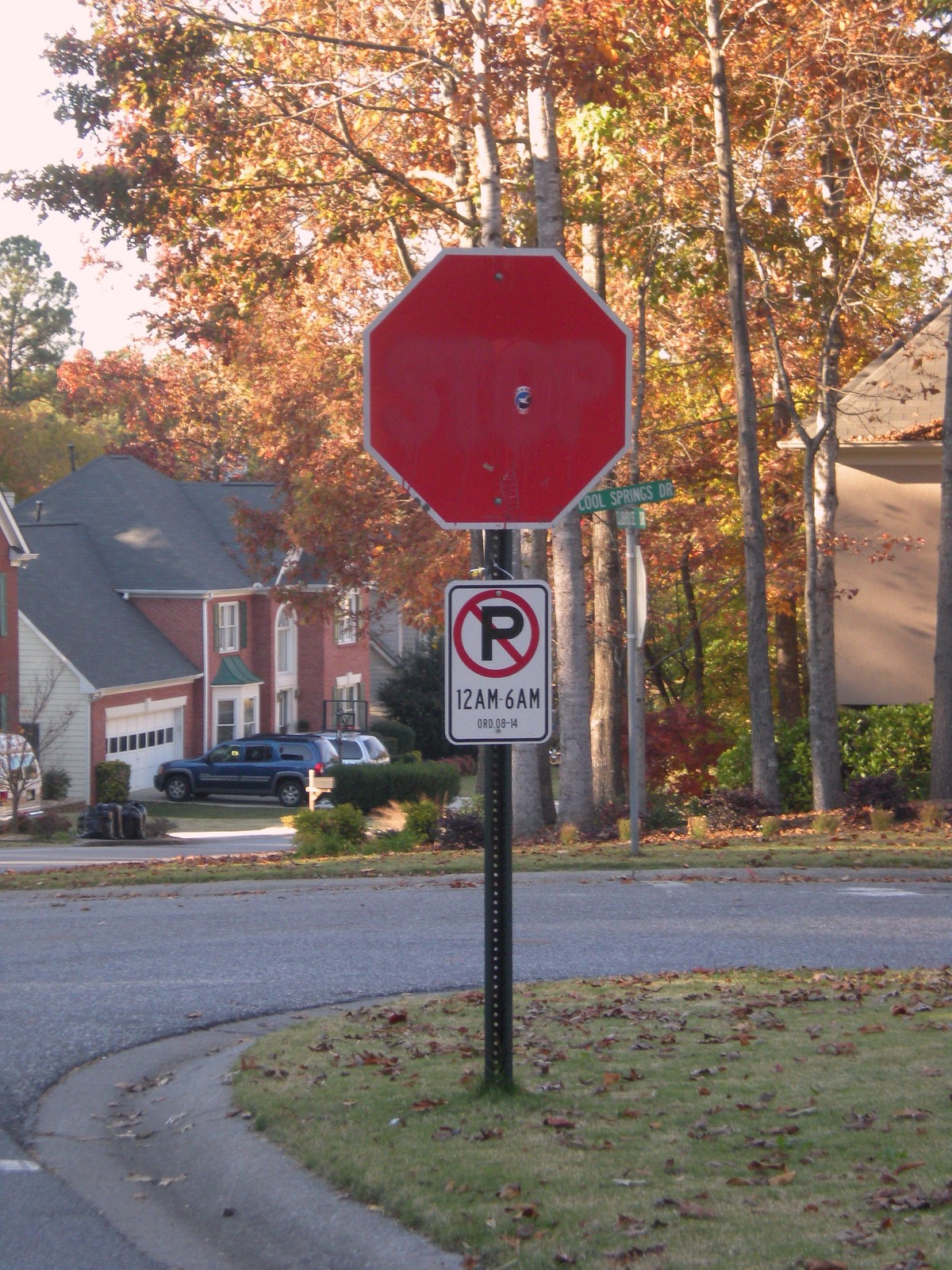In this photograph taken in a suburban neighborhood, we see a stop sign prominently positioned at a street corner. The stop sign is notably unusual as its white lettering seems to have been either faded or spray-painted over, leaving only a faint, barely visible imprint of the word "STOP" against the red octagonal background with a white border. The sign is mounted on a typical green metal post with perforations along its center. Below the stop sign, there is a smaller white "No Parking" sign featuring a black "P" crossed out by a red circle and diagonal line. This sign specifies "12 a.m. to 6 a.m." and includes an ordinance number "ORD 08-14".

The signpost stands in a grassy area that forms a median along a curved roadway, suggesting the location might be near a roundabout or a bend. Surrounding the scene is a well-maintained neighborhood with no visible parking. Across the street, a large, beautiful brick house with a white garage and a drive-up parking area is visible. The neighborhood appears affluent and is marked by a street sign naming it "Cool Springs Drive."

Adding a touch of seasonal ambiance, the trees scattered throughout the background exhibit a vibrant mix of green, yellow, and orange leaves, indicative of the fall season. Fallen leaves adorn the grassy patches, and a partially visible sky peeks through the foliage, completing the picturesque suburban setting.